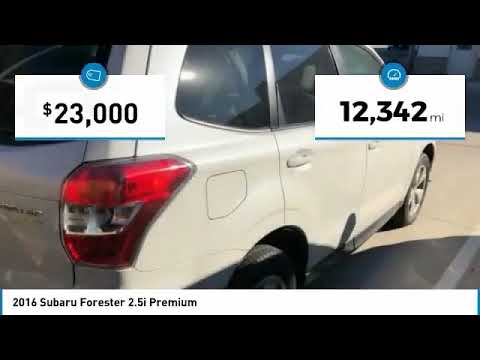The image is an advertisement for a 2016 Subaru Forester 2.5i Premium, featuring a photograph of the car parked, showing mainly its right-hand side and back end. The car is white with black tires, visible red taillights, and shadows cast by the sun. It's positioned within an ad bordered by large black bars at the top and bottom. A secondary white bar between the car and the bottom black border displays the model information in black font. In the upper left corner, a blue icon with a price tag is depicted, showing "$23,000" in black text within a white box. Similarly, in the upper right corner, an odometer icon indicates "12,342 miles" in black text within a white box. Despite the close-up view of the SUV, which appears to be parked in a lot or designated space, the car’s condition cannot be definitively assessed.